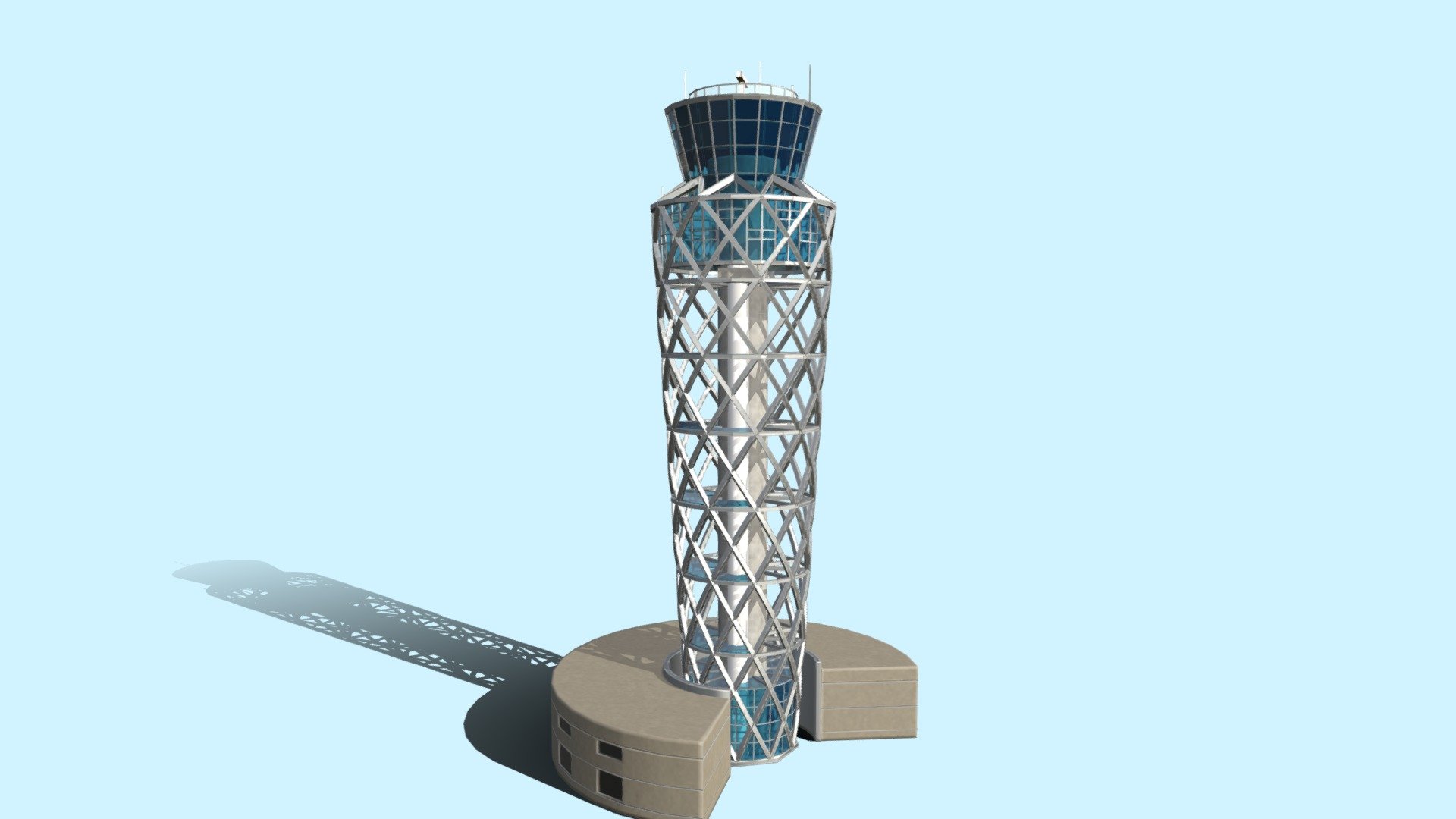The image depicts a detailed 3D rendering or CAD illustration of an air traffic control tower set against a light bluish-green background, likely intended for an instructional manual or architectural review. The base features a two-story, C-shaped beige building with two rows of windows approximately every 15 feet. Centrally located within the C-shaped base is a robust core structure, possibly housing an elevator or stairwell, surrounded by an intricate crosshatch or honeycomb-like metal framework. The tower extends upwards to a glass viewing area at the top, resembling the crown of a torch, with a gradient of blue windows transitioning from dark to light. A small antenna and a white shape are positioned at the very top of the tower, casting a shadow to the left, adding to the realistic detail of this illustrative model.